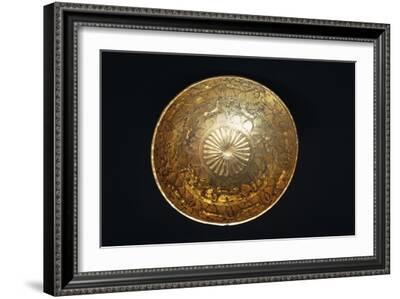The image features a horizontal rectangular black picture frame with a smooth exterior accented by small, decorative dots along its edge. Inside the frame, which is slightly tilted with the left side appearing closer to the camera, there's a light gray shadow behind it on the left, adding depth. The frame is bordered on the inside by a beige, cardboard-like matting. Within this matting, a central black background showcases a round, bronze-colored medallion with intricate, ornate carvings. This medallion, possibly a bowl or shield, features radiating lines and curves that converge on a small central indentation, adding texture and depth to the object. The arrangement of the image and its shadows create a 3D effect, drawing attention to the detailed craftsmanship of the bronze centerpiece.